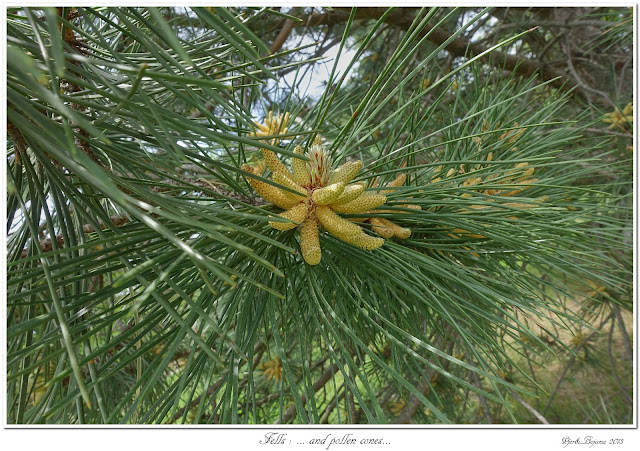In this detailed photograph set in a lush, tropical environment, the focus is on the vibrant natural elements, particularly featuring a blooming pine tree. Central to the image is a cluster of long, yellow-orange pollen cones emerging conspicuously from the heart of the tree, amidst an abundance of lush green vegetation. The backdrop includes verdant grass transitioning to patches of browning areas, painting a picture of the ground beneath. The sky overhead is partly cloudy, revealing glimpses of blue peeking through, with clouds scattered gracefully across. Surrounding the central pine tree, characterized by its elongated green needles and light gray branches, the panorama extends to more distant trees and foliage. The image, devoid of any text save for a small caption at the bottom indicating "fells and pollen cones" along with a date stamp from 2013, captures the dynamic and colorful palette of green, brown, yellow, orange, red, tan, and black, effectively encapsulating the richness and vitality of the tropical scene in broad daylight.